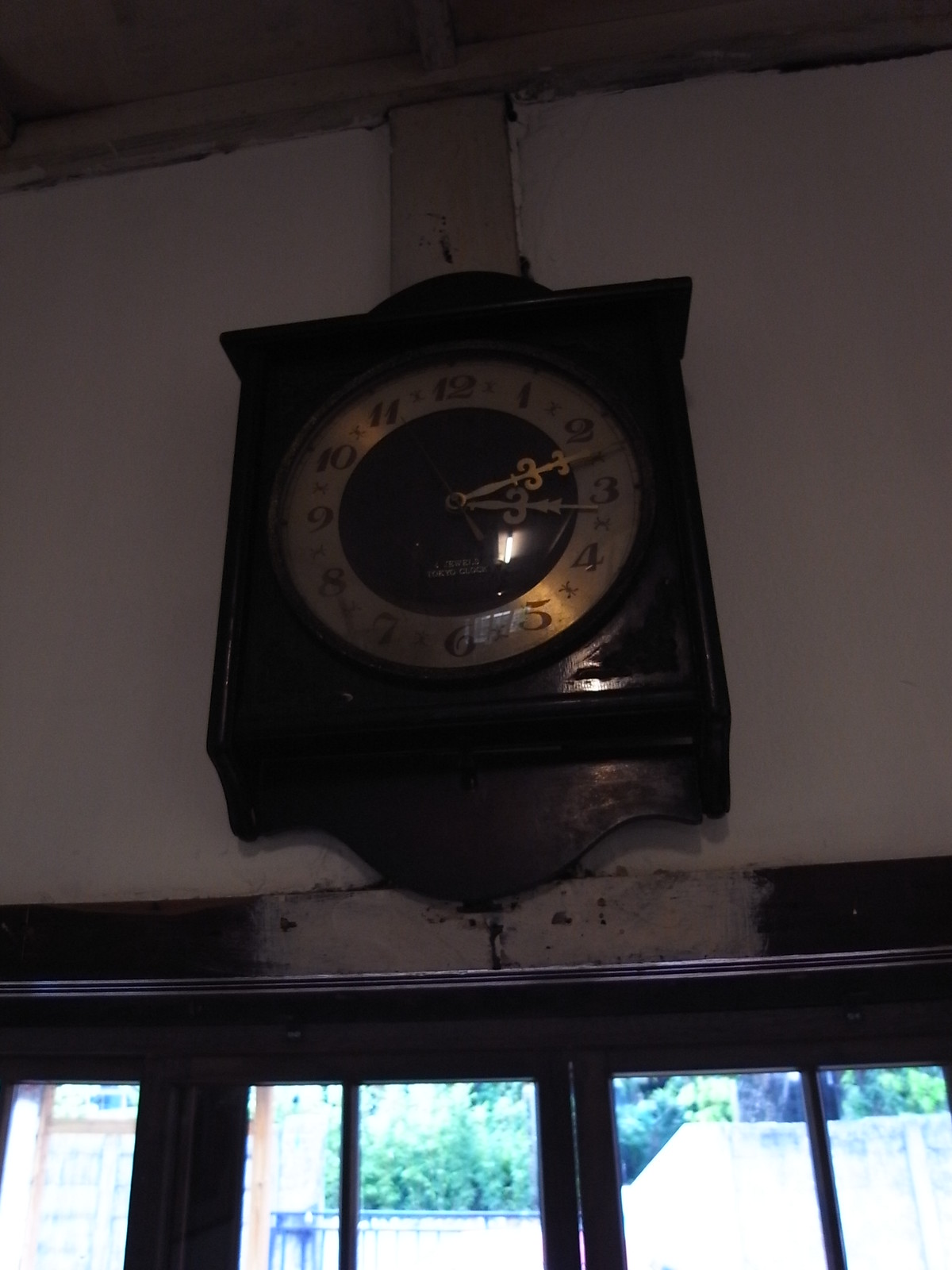The image depicts an antique, square-shaped wooden clock mounted on an off-white wall, centered on a tan vertical beam. The clock features a dark circular face with a light gold band encircling light brown numbers (1 through 12) with tiny symbols in between. The clock's hands, including the second hand, are gold, and the time displayed is 3:12. Centered above the clock face is a semicircular design, complemented by a wavy pattern beneath. Beneath the clock, a dark trim, possibly grayish or whitish in certain sections, outlines the frame of glass windows or doors that allow a view to the outside. The exterior scene reveals trees and shrubbery, suggesting a clear day. Noteworthy is the patch of white paint on the middle section of the trim directly below the clock, further emphasizing the clock's antique aesthetic.